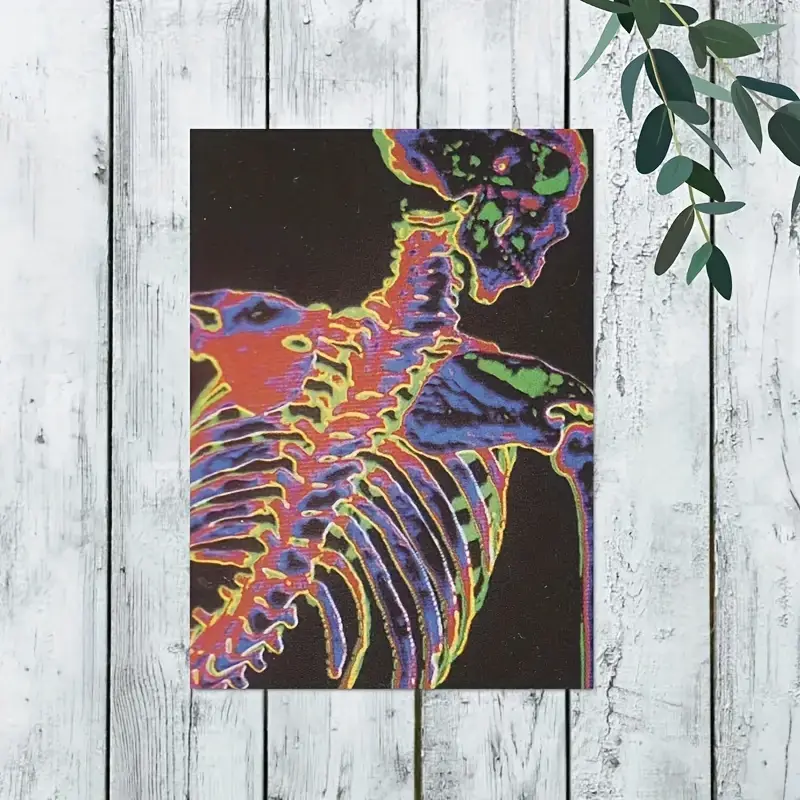The image showcases a vibrant, handmade painting of a partial human skeleton on a black canvas, attached to a white painted wooden fence outdoors. The skeleton, arranged diagonally from the bottom left to the top right, is vividly colored with hues of purple, red, blue, green, and yellow. It features the skull, rib cage, spine, and parts of both arms, with the right shoulder specifically highlighted in red. The skeleton is seen in profile and positioned such that it adds a dynamic flow to the composition. In the top right corner of the photograph, a sprig of leaves is visible, adding a natural element to the scene. The overall image is well-lit, emphasizing the brightness and details of the colorful painting.